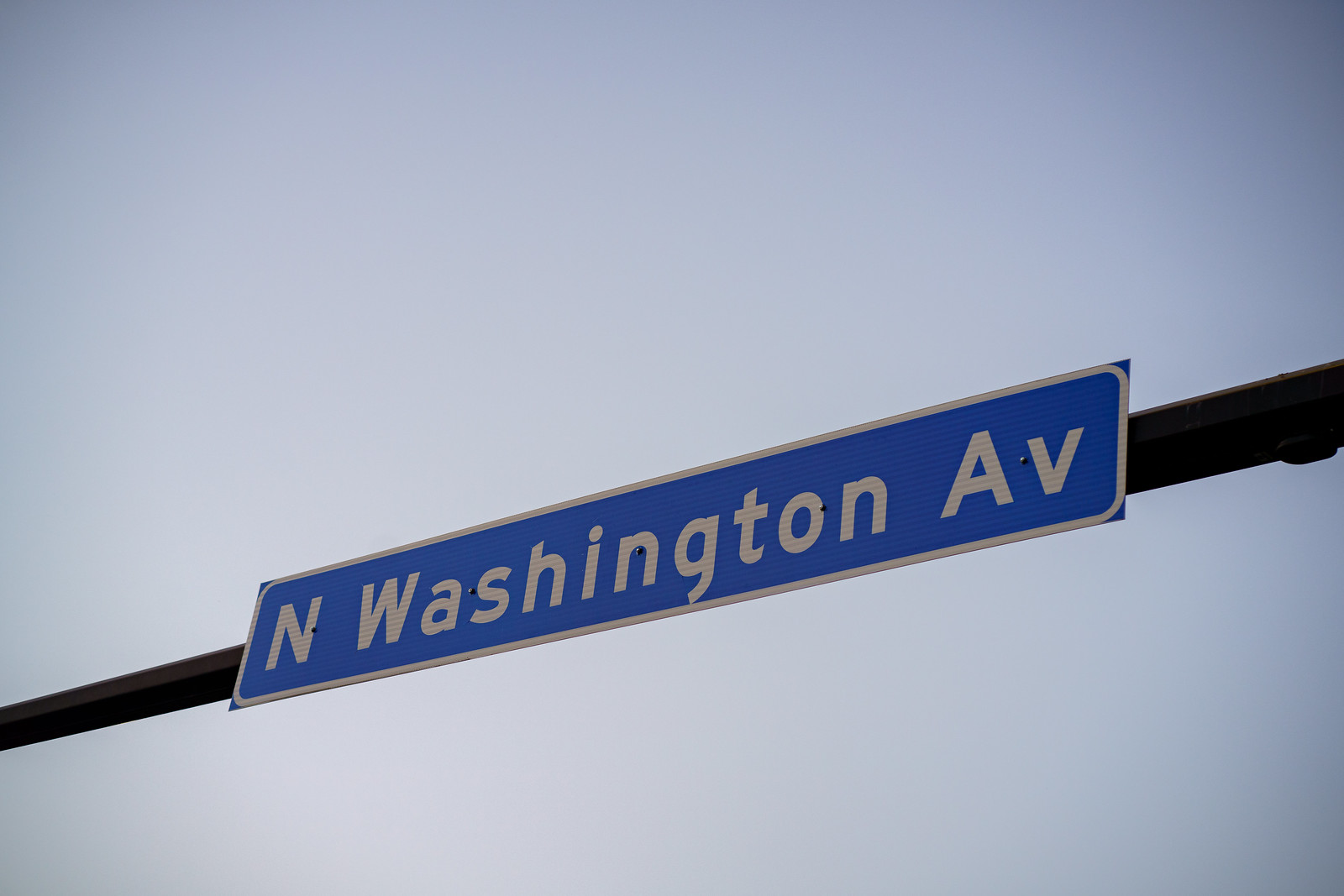This close-up photograph features a street sign against a blue-gray sky. The street sign is captured with meticulous detail, positioned primarily within the center of the frame. A thick black line extends horizontally across the photograph, slightly slanting upwards towards the right. About a quarter of the way up from the bottom on the left-hand side, the line begins and ascends, creating a subtle diagonal effect.

At the forefront of this line lies a prominent blue rectangle with a white outline, clearly distinguishing the sign from the background. The sign bears white lettering that spells out "N. Washington A.V." The sky in the background exhibits a gradient of slate blue-gray hues, with darker tones concentrated in the right corners, both top and bottom, framing the sign in a moody, atmospheric light. This contrast accentuates the street sign's colors and details, giving it a striking appearance against the serene, muted sky.